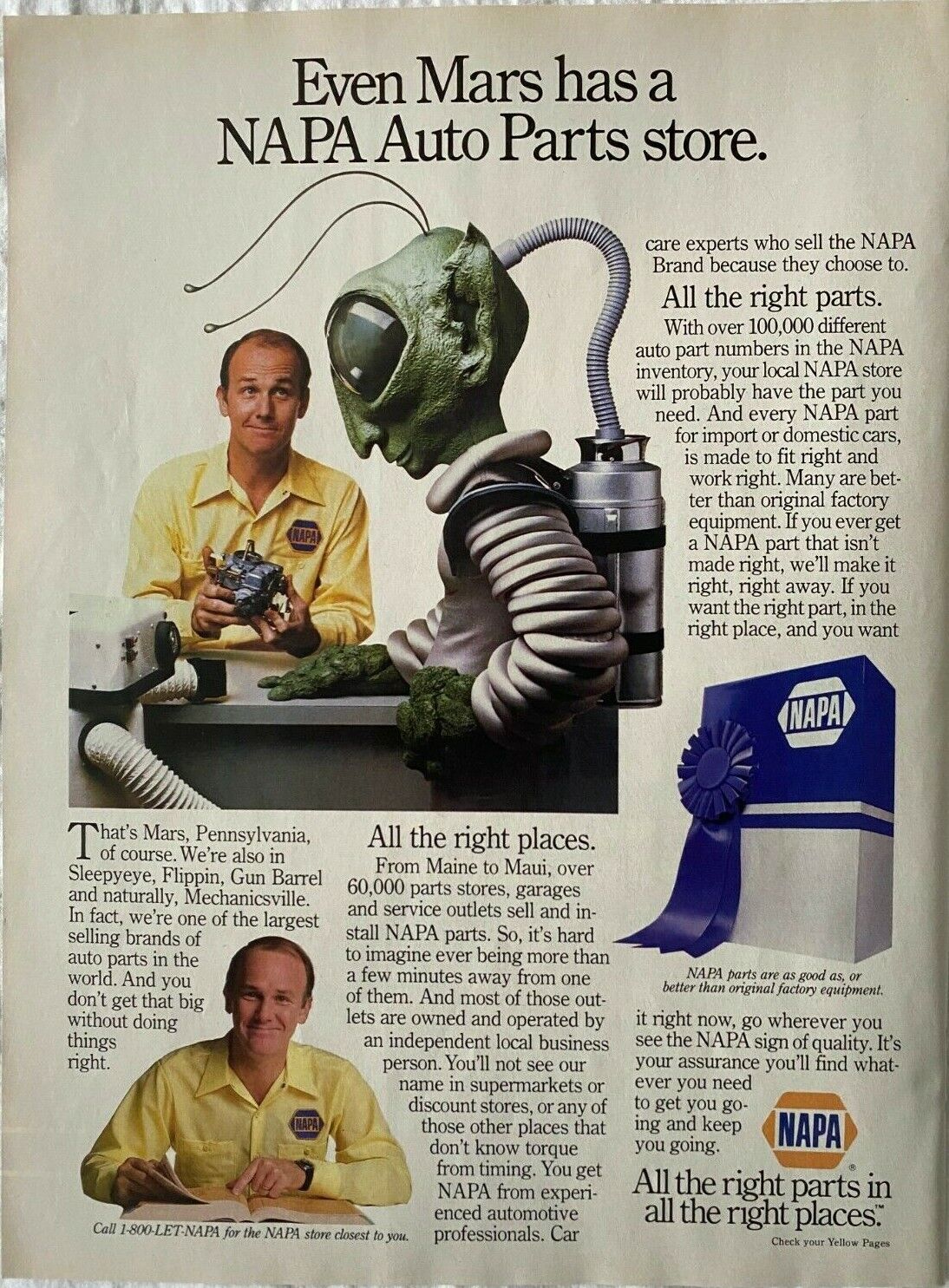This image is either a scanned page or a photograph from an illustrated book or publication. The page features a clean white background with prominent serif text at the top that reads, "Even Mars has a NAPA Auto Parts store," with "NAPA" in all capitals. Below this heading, on the left side of the page, there is a visually engaging photo illustration. This illustration depicts a large alien figure with an oversized head, characterized by two prominent antennas and large expressive eyes. The alien is equipped with a peculiar pipe-like apparatus extending from the back of its head to a cylindrical device on its back. The alien stands confidently with one hand on its hip and the other resting on a counter next to a NAPA Auto Parts store employee, identifiable by their yellow shirt. Within the scene, a robot is also positioned to the left of the alien, adding to the otherworldly ambiance.

At the bottom of the page, there is another photograph of a NAPA employee, the same individual depicted in the aforementioned illustration. This employee is wearing the signature yellow shirt and is seated at a desk with an open book, smiling warmly at the camera. On the right side of the page, there is a detailed image of a blue and silver box. The top portion of the box is royal blue and proudly displays the NAPA logo in white, accompanied by a blue ribbon, emphasizing the brand's identity.